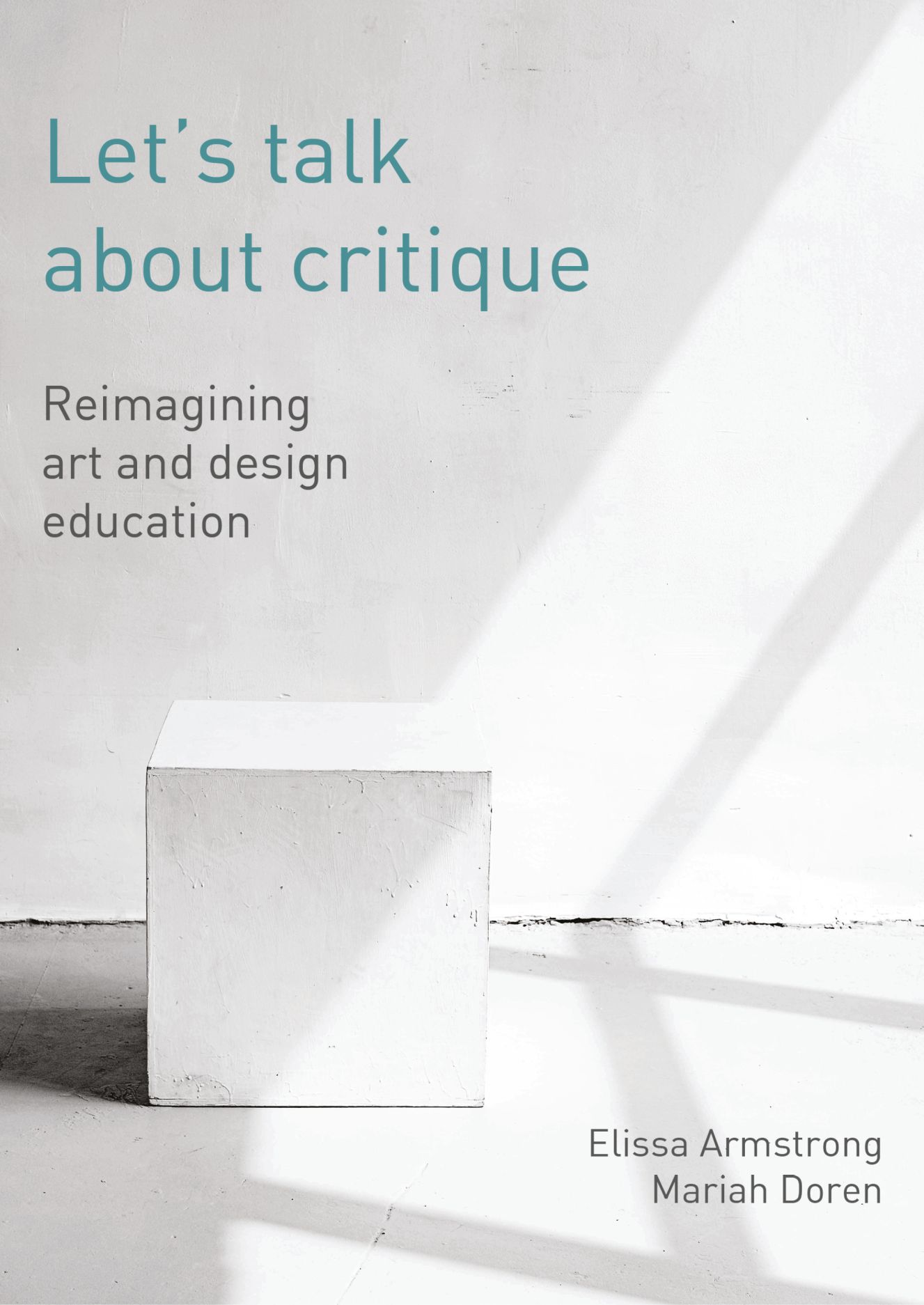This image features a minimalist, white-walled room with a concrete floor, both surfaces showing signs of cracks where they meet. Sunlight streams in from a window out of frame on the right, casting shadows of window crossbeams across the scene. Central to the composition is a plain, white cube that sits slightly off-center to the left. In the upper left corner of the image, teal text reads, "Let's talk about critique," followed below by black text stating, "Reimagining Art and Design Education." In the bottom right corner, the names "Alyssa Armstrong" and "Mariah Doran" are written in black, likely indicating the speakers for the event.